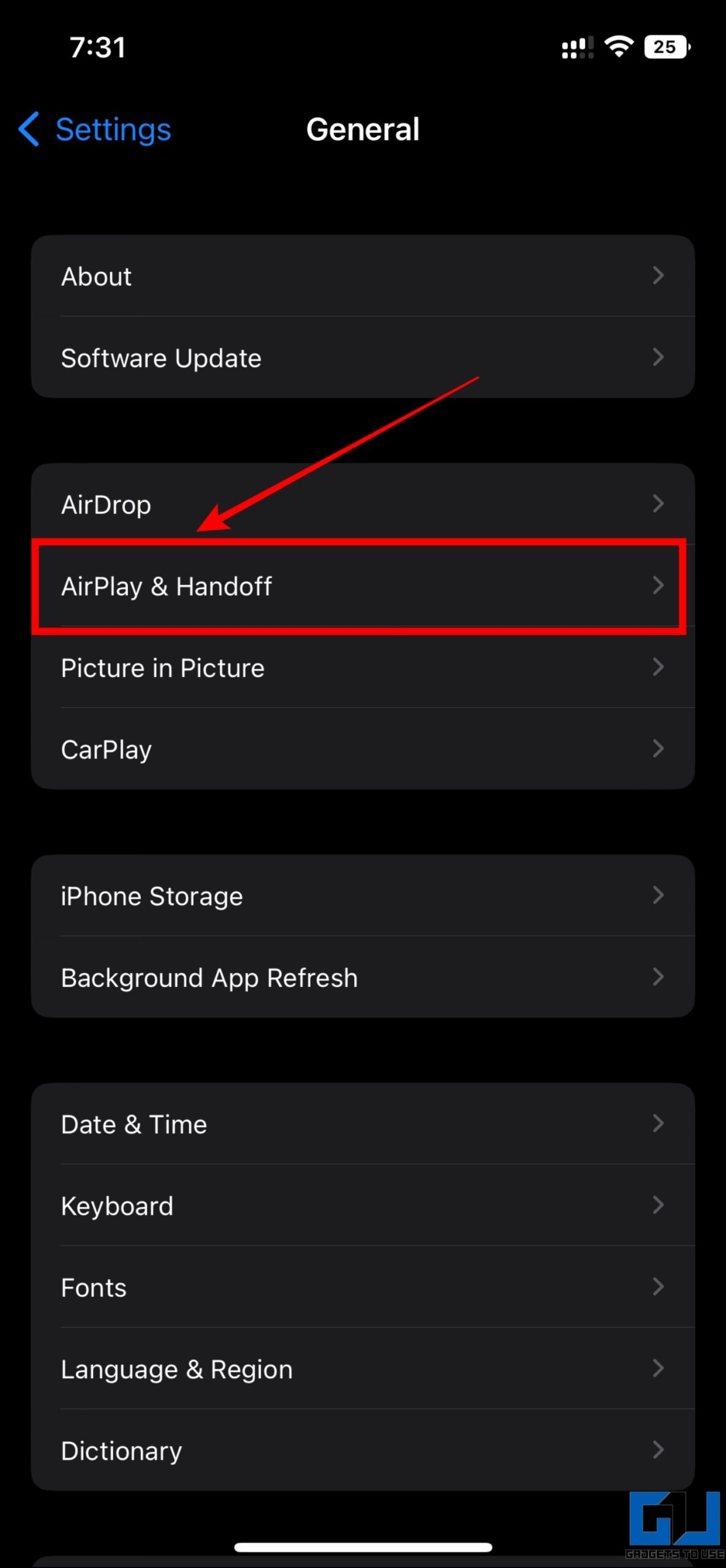This image is a screenshot captured on an iPhone displaying a section of the device's Settings under the General category. The time displayed in the top left corner of the screen is 7:31, and the battery icon in the top right corner indicates a 25% charge. The screen is in dark mode, with a black background and white text.

In the top center, the title "General" is clearly visible, confirming the section of the Settings being viewed. On the top left, the word "Settings" is written in blue, accompanied by a blue back arrow pointing left, indicating navigation options within the Settings app.

The content on the screen lists a variety of settings options in a vertical menu. From top to bottom, these options include:
- About
- Software Update
- AirDrop
- AirPlay & Handoff (highlighted with a red outlined rectangle and a red arrow pointing toward it)
- Picture in Picture
- CarPlay
- iPhone Storage
- Background App Refresh
- Date & Time
- Keyboard
- Fonts
- Language & Region
- Dictionary (positioned at the very bottom of the list)

The focal point of the image is the AirPlay & Handoff option, which is emphasized with a red outlined rectangle and a red arrow, suggesting that this setting is of particular interest or importance in the screenshot.